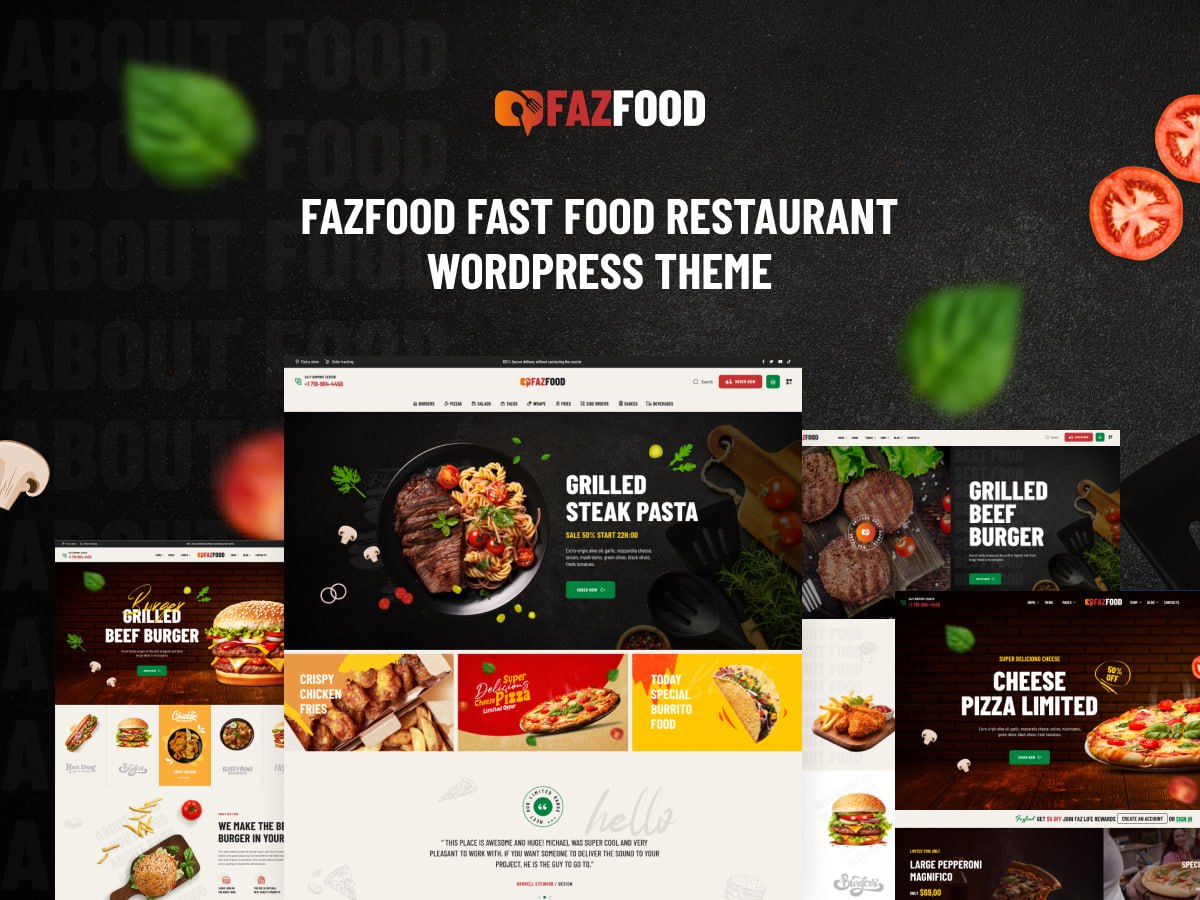Here is a detailed and cleaned-up version of the caption:

---

This image appears to be a screenshot from a website, likely a template for a food-related site. The top section features a black background adorned with slightly blurry images of leaves and halved cherry tomatoes, adding a natural and fresh look. Below, the site showcases various web screens displaying different food items. 

Prominently in the center, there is a section titled "Grilled Steak Pasta," showcasing a delectable dish of pasta with pieces of grilled steak arranged beside it against the same black background. Below this, there are more images and text, although the text is too small to read clearly.

On the right side, there are distinct sections highlighting "Grilled Beef Burger" and "Cheese Pizza Unlimited," each accompanied by appetizing images of these dishes. Another section at the bottom shows an image of a burger with what appears to be fries, though the text is illegible.

On the left-hand side, another section features "Grilled Beef Burger" again with an accompanying image, followed by a white area filled with various food images, showcasing the diversity of offerings.

Further examining the lower part of the screenshot, the text reads, "This place is awesome," and mentions a person named Michael, described as super cool and very pleasant to work with, suggesting his capability to deliver sound for projects—a curious inclusion for a food website. The topmost section states "fast food, fast food, fast food restaurant, WordPress theme," indicating that the image is likely from a WordPress template designed for fast food restaurants.

---

This caption provides a clear and detailed description of the content and layout of the website screenshot.